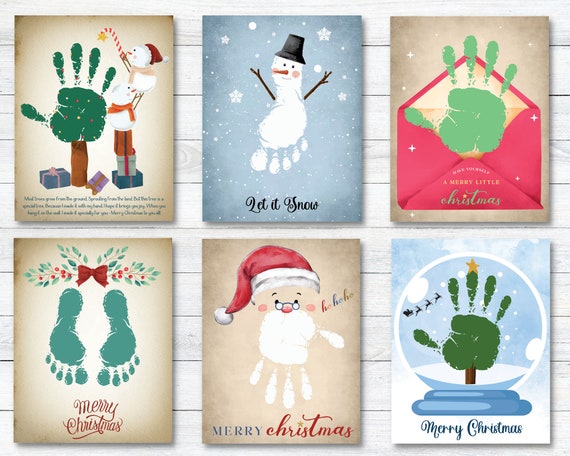This image showcases a collage of six kid-friendly Christmas cards, arranged in two rows of three, photoshopped onto a white-painted wall. Each card creatively incorporates hand or foot prints into festive designs:

1. **Top Left**: A beige card features a green handprint decorated as a Christmas tree on a wooden stump, with a smiling snowman placing a yellow star atop the handprint while standing on three blue presents.

2. **Top Center**: A blue card displays a snowman with a white footprint as its body, adorned with a black top hat, carrot nose, twig arms, and surrounded by snowflakes, with the text "Let it Snow" at the bottom.

3. **Top Right**: A red envelope contains a green handprint resembling a Christmas tree, with three red pieces anchoring the design. The envelope is open, revealing the card inside.

4. **Bottom Left**: A pair of green baby footprints form the base of a festive design, topped with a red bow tie. Above the footprints is a festive wreath with red berries and green leaves, and the card bears the text "Merry Christmas."

5. **Bottom Center**: Santa Claus’s face is crafted from a white painted palm print, complete with glasses, beady eyes, a red button nose, and a classic red-and-white hat. The card says "Ho, Ho, Ho" and "Merry Christmas."

6. **Bottom Right**: A snow globe card features a green handprint Christmas tree with a yellow star on top. Inside the globe, there is a silhouette of Santa and his reindeer against a snowy backdrop, with "Merry Christmas" at the base.

Each card uniquely blends hand and foot prints into charming Christmas themes, making the designs both personal and festive.